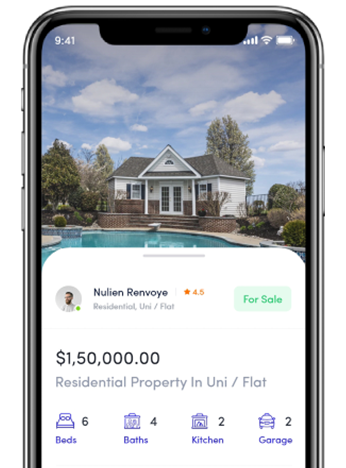This is a screenshot of a cell phone displaying a real estate listing for a house that appears to be for sale. At the top of the phone's screen, there is a photo of the property in question. The house itself is a beautiful white and brick structure that curves around slightly, resembling a ranch-style home. A well-maintained pool with a diving board is visible, though partially obscured by an information box on the screen. Surrounding the house are mature, fully-grown trees, adding to the property's appeal. In the background, a picturesque sky dotted with clouds enhances the overall charm of the scene.

The phone's status bar shows it's 9:41, with visible icons indicating strong Wi-Fi connectivity, full cellular signal bars, and a nearly full battery. Below the photo, a white section with a gray top line features the listing details: the property is labeled under "Nulian Renvoy," categorized as residential, in the "Yuri / flat" area. A green button confirms the house is "For Sale," indicating an asking price of $1,050,000.